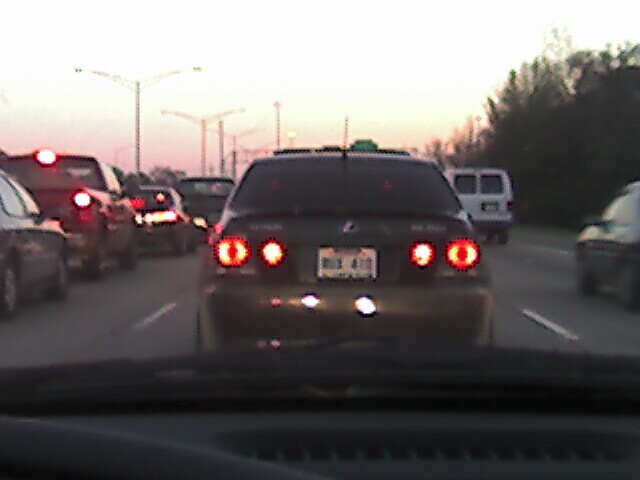In this particular image, captured from a low-quality dashcam likely positioned on the rear-view mirror, we find ourselves sitting in a vehicle in the midst of traffic. Directly ahead is a brown Lexus sedan with four red tail lights, though its license plate is obscured. The scene is bathed in the hues of an evening sunset, with red and yellow tones coloring the sky, and several cars have their full beam lights on, indicating it is dusk. Surrounding our vehicle are various other cars: to the left, there's a mix of pickup trucks and compact cars of different colors, all appearing to be at a standstill; to the right, traffic is slightly more fluid, as evidenced by a white van and another compact car moving swiftly, resulting in a more blurred appearance. The road, spacious and indicative of a western country, possibly America, is lined with several vehicles all seemingly caught in a moment of shared stillness.